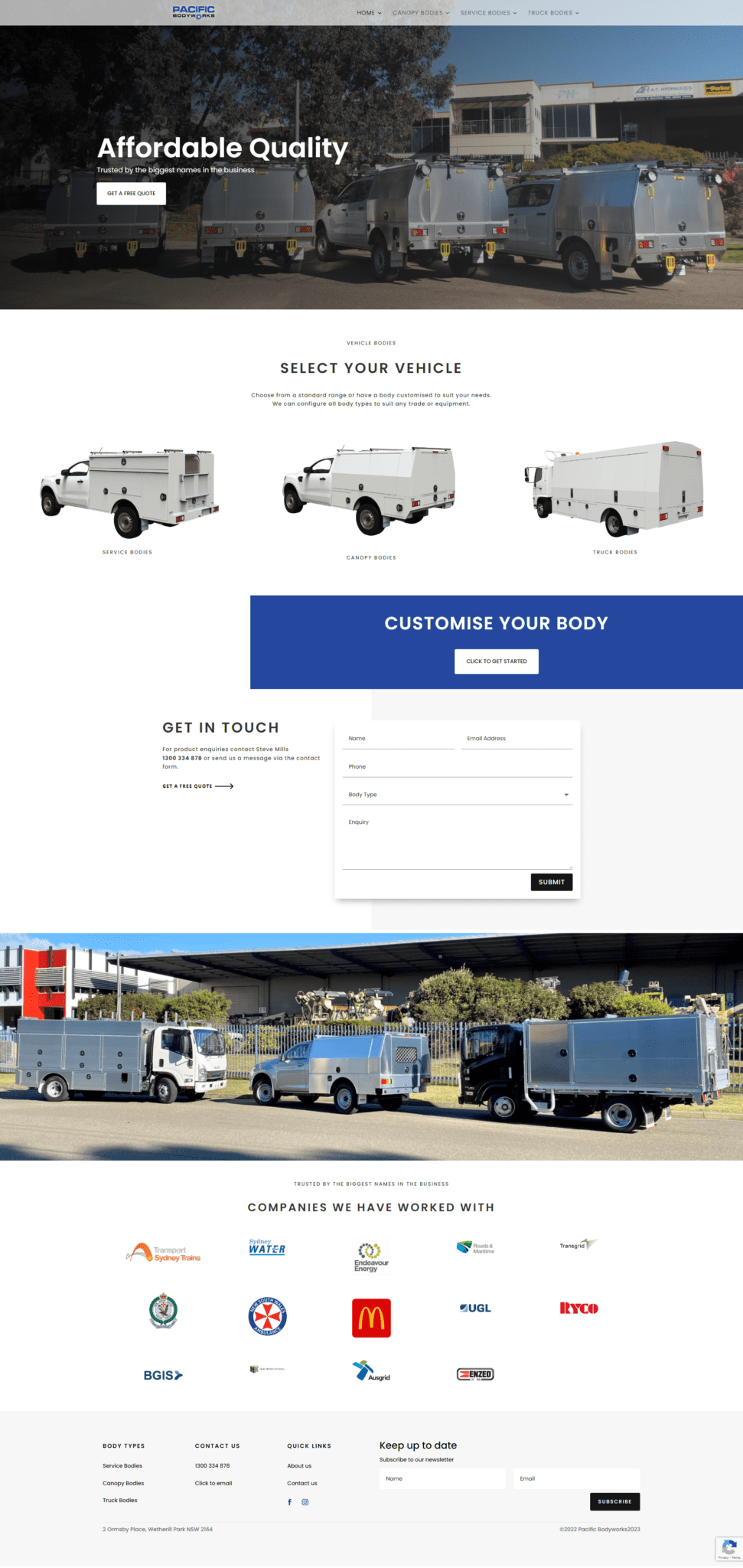The image features a webpage with a gray border at the top, containing some small, unreadable text. At the top of the page, there is a picture depicting four work trucks parked in front of a building, with trees and a blue sky in the background. The image bears the text "Affordable Quality" and includes a clickable white button beneath it. Below this, there is the heading "Select Your Vehicle," accompanied by images of three different types of white trucks, each with distinct features. A blue box labeled "Customize Your Body" is shown underneath. Further down, another picture is displayed, featuring three trucks of varying sizes parked in a lot, also set against a backdrop of trees, a building, and a blue sky. At the bottom of the page, a list of corporate sponsors is visible, with McDonald's being the only recognizable name.